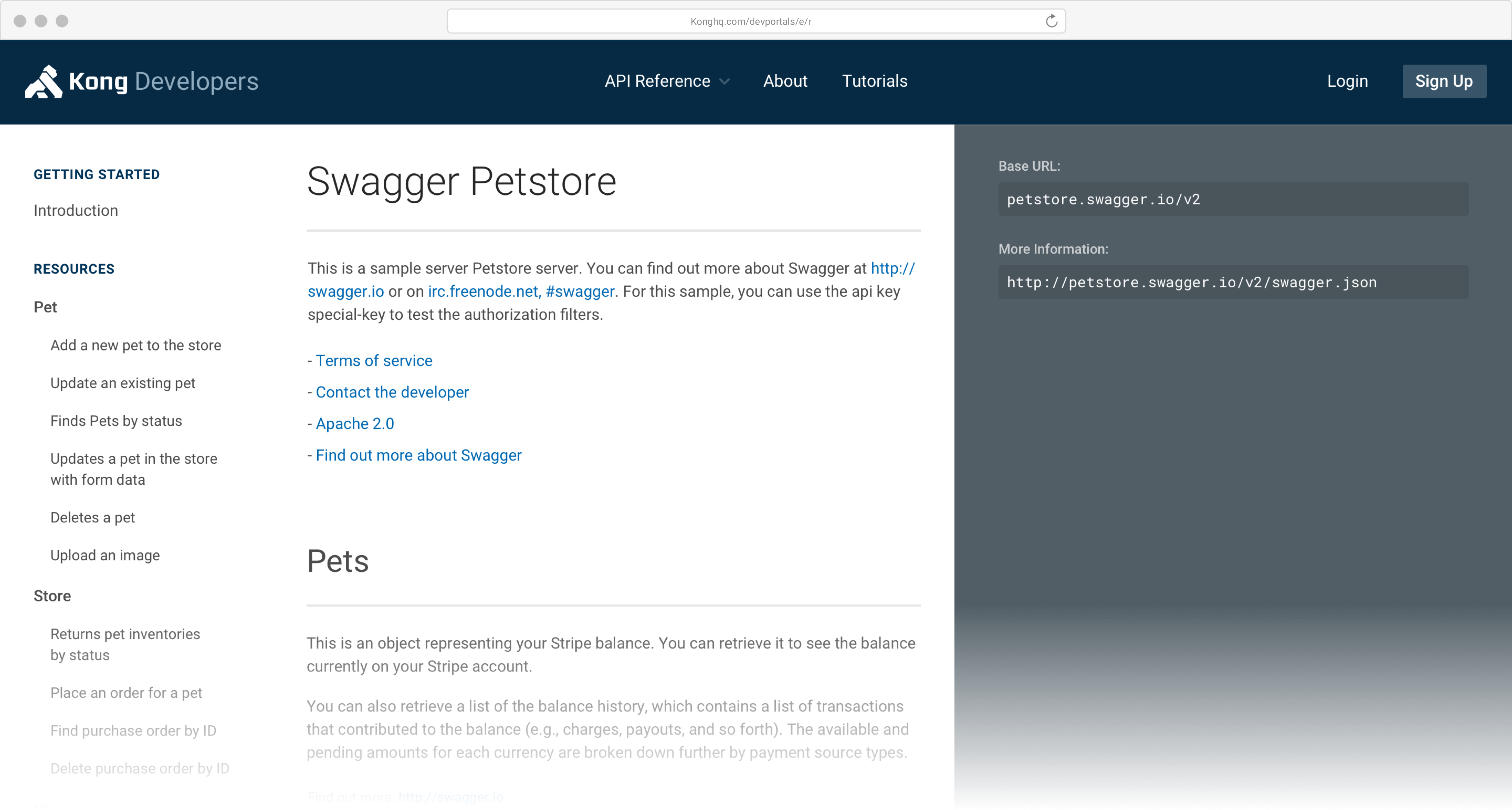This is a detailed screenshot of the Kong Developers website interface. The top of the page features a prominent blue navigation bar extending horizontally. On the left side of this bar, "Kong Developers" is displayed, with "Kong" in white text and "developers" in gray. Centrally positioned within the navigation bar are three buttons labeled "API Reference," "About," and "Tutorials," all in white text. The "API Reference" button includes a dropdown menu. On the right side of the navigation bar are "Log In" and "Sign Up" buttons, with the latter being a gray, box-shaped button.

Beneath the navigation bar, the content is organized into three columns. The left column serves as a sidebar, listing various sections such as "Getting Started," "Introduction," "Resources," and multiple functions related to pets, including "Add a New Pet to the Store," "Update Existing Pet," "Find Pets by Status," "Update a Pet in the Store with Form Data," "Delete a Pet," and "Upload an Image."

In the central column, a headline prominently reads "Swagger Pet Store," followed by a subheading that states, "This is a sample server pet store server." This central area appears to be the main content section, providing an overview and context for the website's functionalities. The right column's contents are not described in the screenshot narrative. The overall layout is clean and organized, presenting a user-friendly interface for accessing various developer resources and API functionalities.